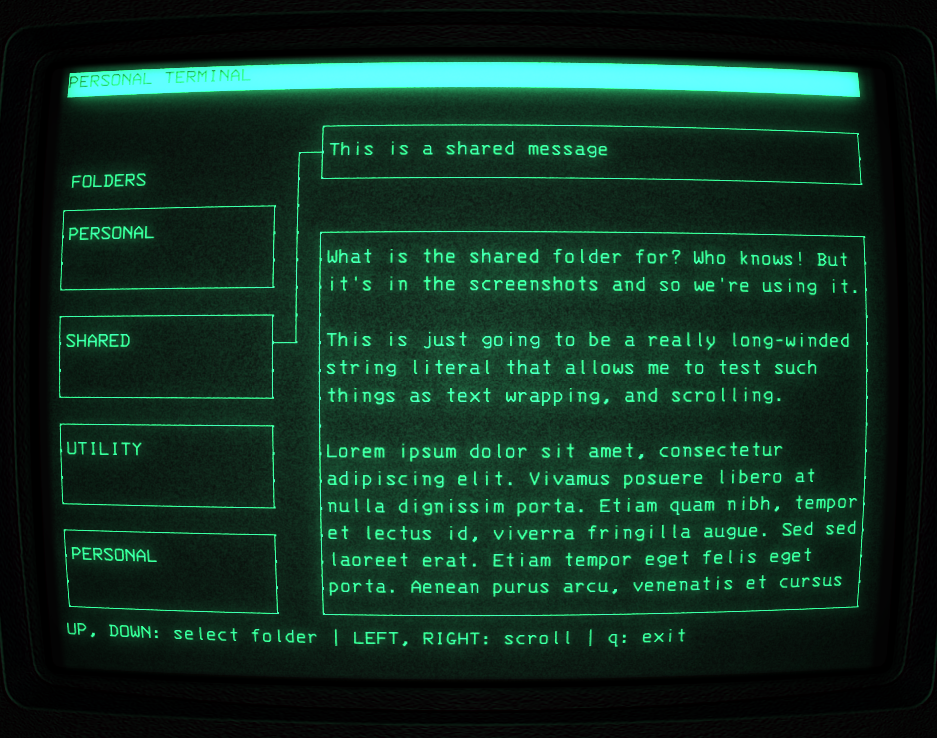The photograph showcases an old computer screen using a green-on-green color scheme, reminiscent of DOS systems. In the very upper left corner, the screen displays "Personal Terminal" on a bright green background. Below that, on the left side section, there is a label "Folders" with four stacked rectangles labeled "Personal," "Shared," "Utility," and again "Personal." A line extends from the "Shared" rectangle to another rectangle that states, "This is a shared message."

In the center of the screen, a large rectangular text box contains three paragraphs. The text reads, "What is the shared folder for? Who knows? But it's in the screenshots, so we're using it. This is just going to be a really long-winded string literal that allows me to test such things as text wrapping and scrolling." The rest of the paragraph contains Lorem Ipsum text.

At the very bottom of the screen, user instructions are provided: "Up, Down, Select Folder, Left, Right, Scroll, Q, Exit." The entire setup appears to be an interface for testing text display and navigation features, possibly used for coding or early computer usage illustrations.